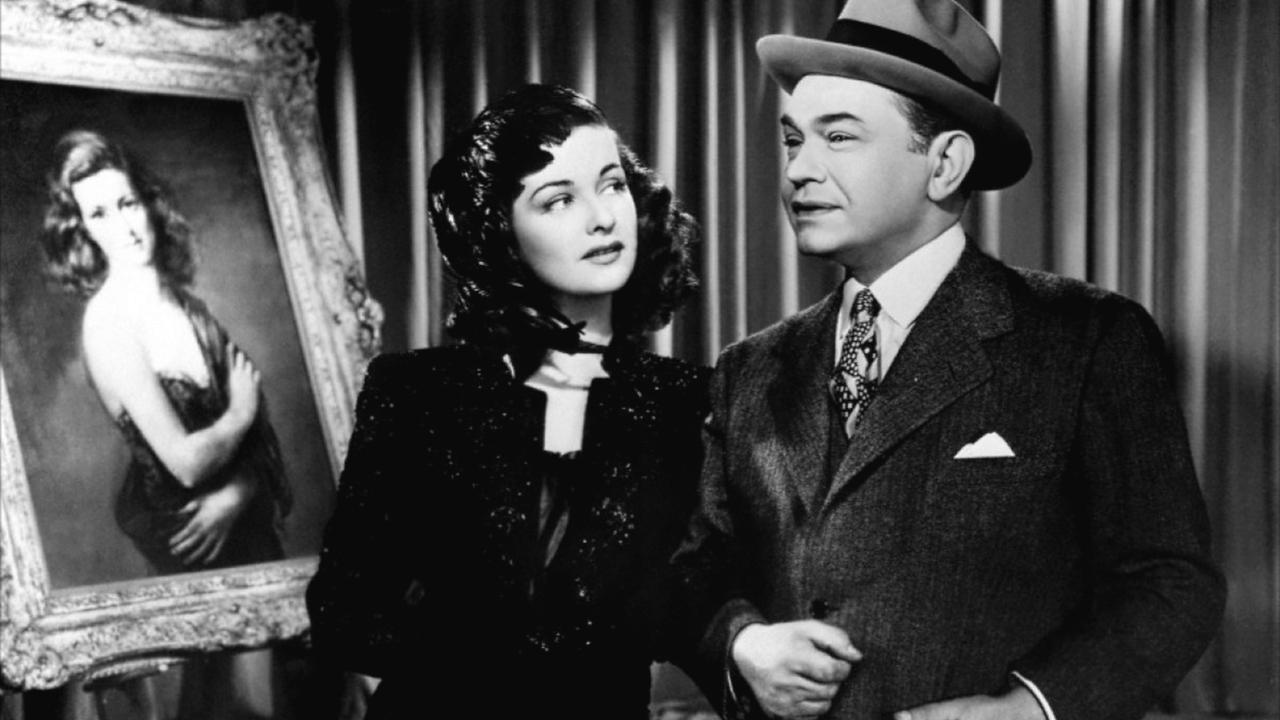This black and white photograph, likely from the 1930s or 1940s, features two individuals—a woman and a man—against the backdrop of thick theater curtains. The woman, dressed in a dark outfit with her hair pulled back, gazes longingly at the man beside her. Her attire, difficult to discern in detail due to the monochromatic nature of the image, appears elegant and possibly comprises a jacket over a dress. The man, sporting a suit and tie adorned with a white handkerchief in the pocket and wearing a hat, stands with his arms folded in front of him.

In the left-hand side of the photograph, there is an ornate picture frame containing an image of another woman, who appears poised and classy in a fancy dress, possibly holding her arms in front of her. This framed woman, with styled hair, adds an element of intrigue and sophistication to the scene, suggesting she might be posing as a model or an actress. The overall composition and style give the impression of an old movie still, encapsulating a bygone era's elegance and charm.